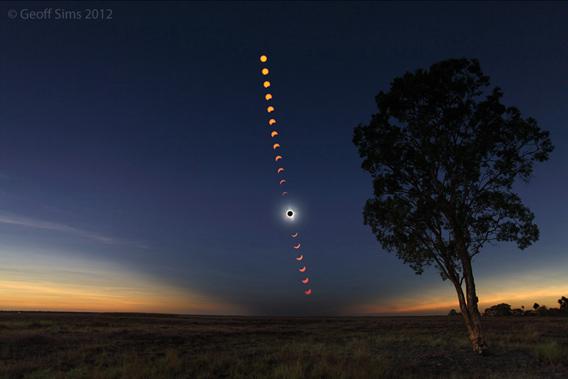In this captivating time-lapse photograph by Geoff Sims from 2012, the serene beauty of a solar eclipse unfolds over a vast, mostly empty field. Taken low to the ground amidst the grass, the image captures a dark evening scene dominated by a singular medium-sized tree to the right, its foliage appearing dark against the night sky. Stretching across the center of the photograph from top to bottom, the solar eclipse is depicted in various stages, each phase marked by different coverings of the moon's shadow over the sun. The sequence begins with yellow-orange dots that gradually deepen into dark orange hues, eventually transitioning into banana-shaped crescents and culminating in the dramatic full eclipse with a glowing white rim around a dark center. The horizon glows with a subtle sunset of light orange and amber, while the sky above transitions to a deep blue, encompassing most of the image. In the top left corner, the photo is discreetly labeled with "Copyright Geoff Sims 2012", adding a finishing touch to this detailed and immersive depiction of a celestial phenomenon.